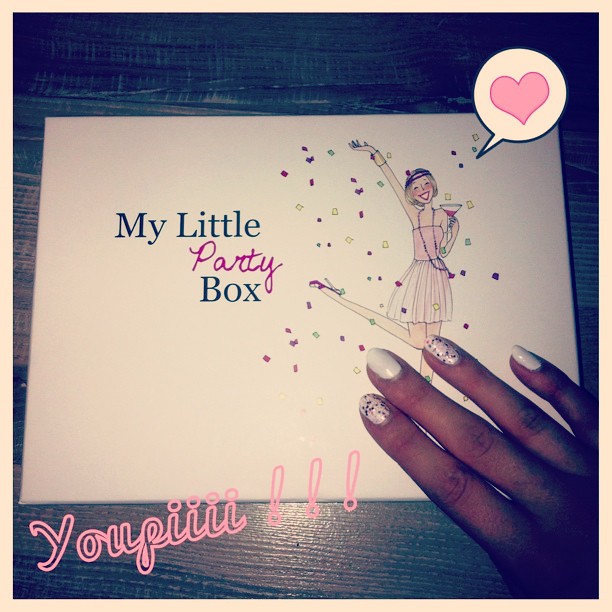The image showcases a white card positioned on a wooden table with a light brown color, artistically enhanced by darker grooves and lines. An overhead perspective captures a hand on the card's lower right corner, displaying white-painted fingernails, with confetti adorning two of the nails. 

Center-left on the card, the handwritten words "my little party box" are scripted, with "party" highlighted in red (or pink, depending on interpretation). The card features an animated illustration of a woman in a dress, striking a joyous pose with one leg raised and arm in the air, holding a cocktail glass. Confetti in vibrant colors such as pink, purple, green, and yellow floats around her. She is accessorized with a purple headband, a purple necklace, pink shoes, and a golden bracelet with a purple charm.

In the upper right, there’s a speech bubble housing a pink heart. The bottom left corner of the image is overlaid with the pink diagonal text "UP!!!!!!" with the exact stylings of "Y O U P" followed by multiple 'I's and exclamation marks. The entire composition is embraced by a cream border, enhancing the festive and playful theme.